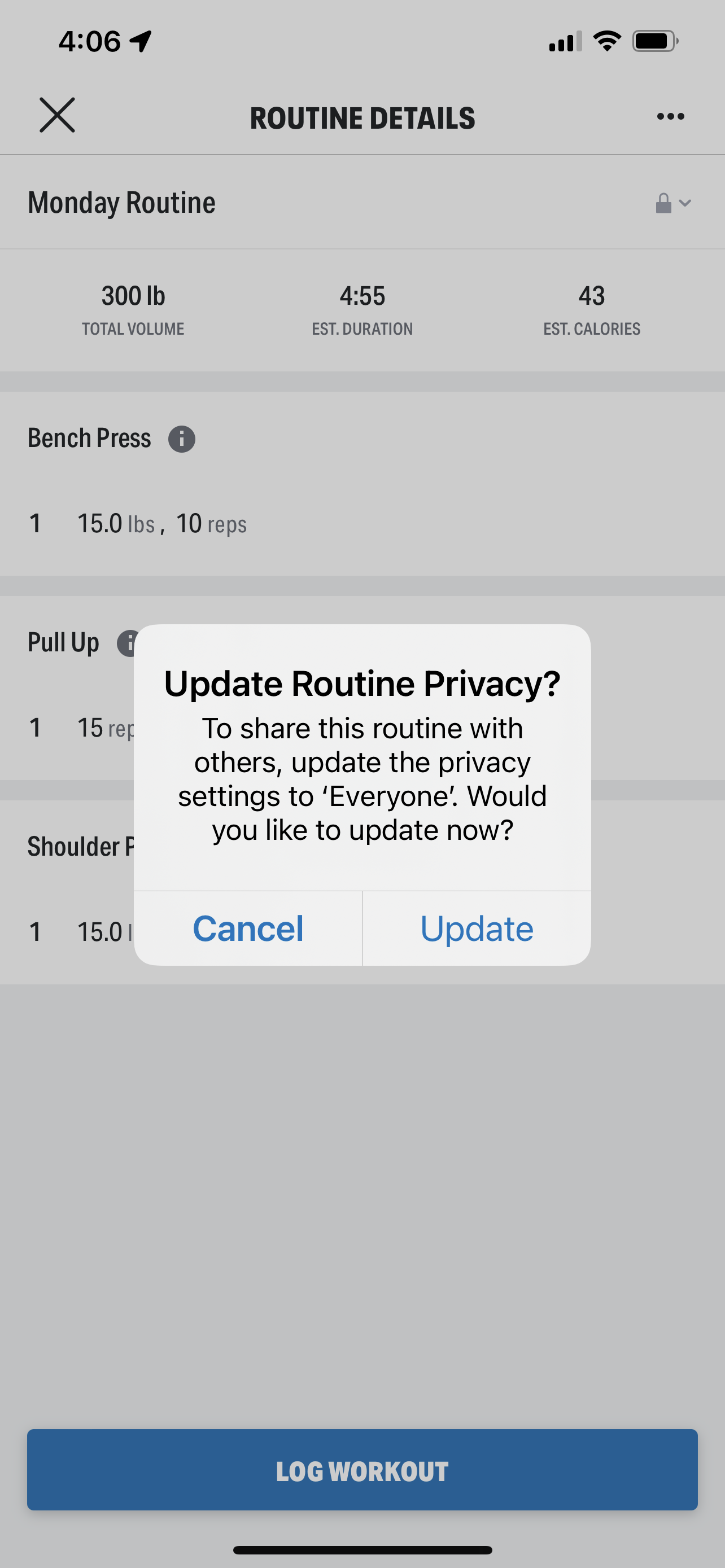In this particular image, we have a screenshot of a fitness app interface. 

At the top left corner, the current time is displayed as 4:06. Adjacent to the time, there are three icons indicating cellular signal strength, Wi-Fi connectivity, and battery life. 

Just below the status bar, there's a "Cancel" icon. Proceeding downward, in bold, capitalized text, "ROUTINE DETAILS" is prominently shown. 

Following that, the text "Monday Routine" appears, indicating the specific routine overview for Monday. Below this header, three key metrics are displayed: 
- "300 lbs" under the label "Total Volume"
- "455 min" for "Estimated Duration"
- "43 kcal" for "Estimated Calories"

Continuing further down, there are three rectangular boxes, each representing a different exercise category:
1. Bench Press
2. Pull-Ups
3. Shoulder Press

Appearing prominently in the middle of the screen is a pop-up message asking, "Update routine privacy?". It further inquires if the user wants to share their routine with others by updating the privacy settings to public. This message includes two action buttons: "Cancel" and "Update", with the "Update" button highlighted in blue.

At the bottom of the screen, another blue button labeled "Log Workout" is visible, providing the option for the user to record their routine.